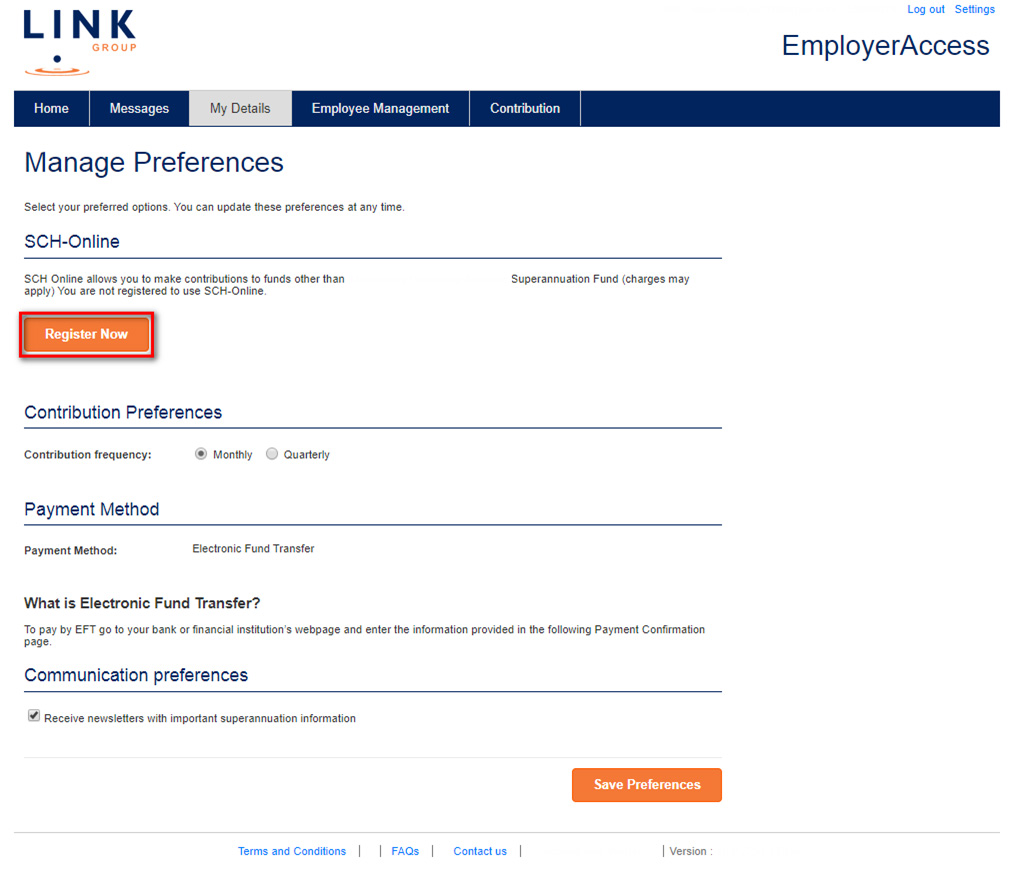The image features a user interface on a white background, primarily divided into multiple sections.

**Top Left Corner:**
- Blue text that reads "Link"
- Below, it says "Group" in the same blue text.
- An icon resembling a blue and white ripple effect, akin to a ball bouncing on water.

**Top Right Corner:**
- Blue text that reads "Logout" and "Settings"
- Directly beneath in very small black text, it says "Employer Access"

**Navigation Bar:**
- A blue line with white text that reads "Home" and "Messages"
- In gray text, it reads "My Details"
- Reverting back to the blue and white theme, it states "Employment Management" and "Contribution" (potentially intended to be "Constitution")

**Main Section:**
- On a white background, blue text that reads "Manage Preferences"
- Black text beneath says "Select your preferred options. You can update these preferences at any time."
- Blue text that says "SCH-Online,” followed by a small blue line.

**SCH-Online Section:**
- Black text explaining "SCH Online allows you to make contributions to funds other than..."
- Followed by an alert in black text stating, "You are not registered to use SCH Online"
- An orange button with white text that says "Register Now"

**Right Side:**
- Blue text stating "Super National Fund" (seems there might be some text missing here)

**Contribution Preferences:**
- Blue text stating "Contribution Preferences"
- Subtext for options: "Contribution Monthly or Quarterly," with "Monthly" checked
- "Payment Method" section explaining the method as "Electronic Fund Transfer"
- Instructions for EFT, stating "To pay by EFT, go to your bank or financial institution’s webpage and enter your information provided in the following confirmation page."

**Communication Preferences:**
- Checkmark box labeled "Receive newsletters with important superannuation information"

**Bottom Section:**
- Bottom left features an orange button with white text that says "Save Preferences"
- Bottom center includes blue text links: "Terms and Conditions," "FAQs," "Contact"
- A section appears whited out
- Black text that reads "Version" followed by a version number

Note: There is an indication that some text at the bottom might be missing or obscured.